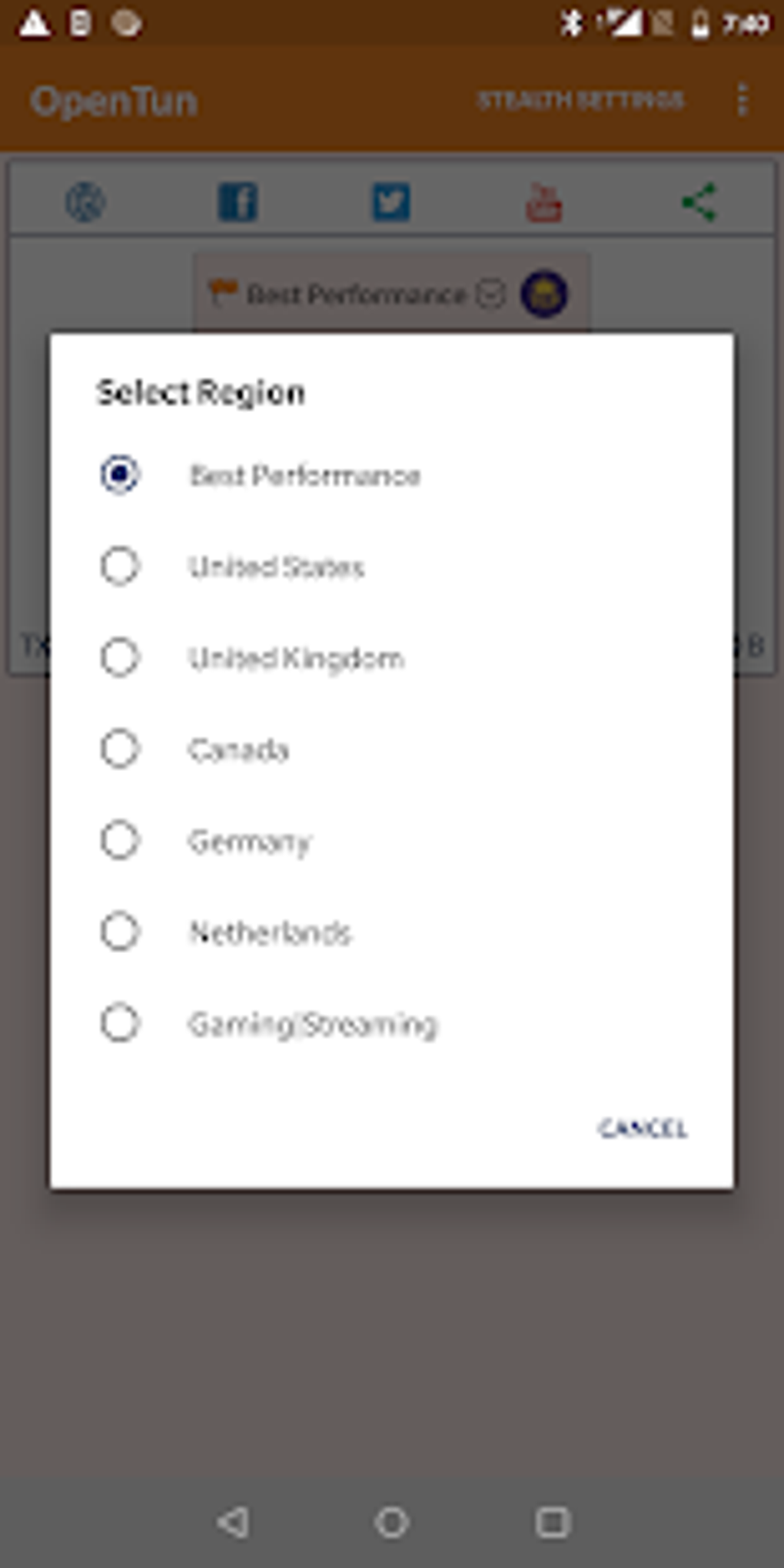The image is a screenshot captured on a smartphone that prominently displays a user interface. The background features an orange bar at the top, which contains essential smartphone indicators such as the battery percentage icon, network signal strength, Bluetooth status, and the current time—though the time is somewhat obscured.

Positioned on the orange bar, the text "Open 10" is visible in white ink. Below this, more white text reads "Settings" and "Search settings." Below the orange bar, there are several application icons displayed in a row: potentially WhatsApp or Google as the first icon, followed by recognizable logos for Facebook, Twitter, Reddit, and a share button.

In the foreground, a pop-up screen with a white background overlays the rest of the interface. This pop-up contains the text "Select Region" prominently at the top. Below this heading, there are several regions listed in black ink, but the names are not clearly visible. The pop-up also features a "Cancel" button located at the bottom right corner.